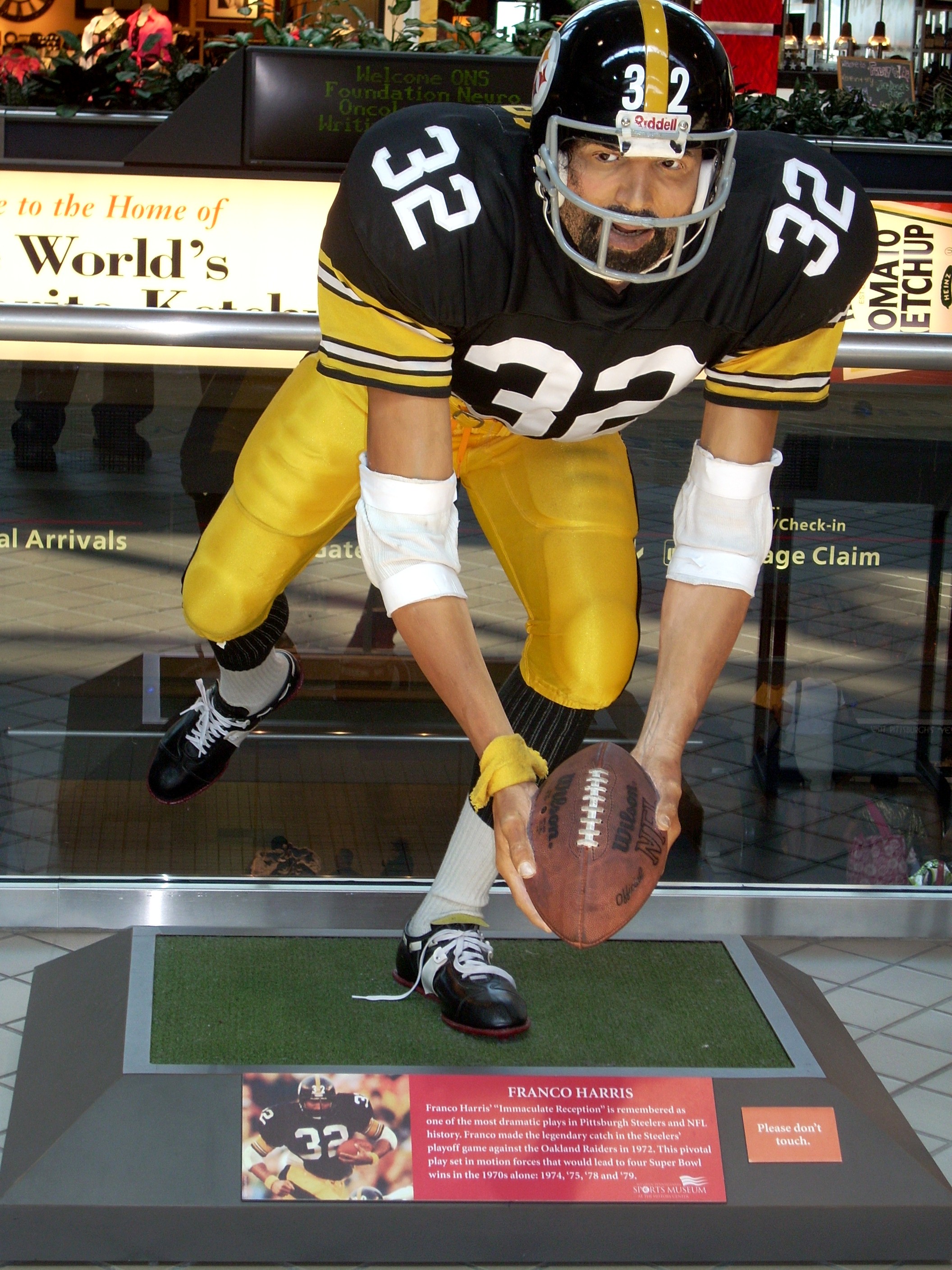This color photograph captures a highly realistic wax figure of Franco Harris, a professional football player celebrated for his legendary "Immaculate Reception." The life-like statue stands in mid-play, with one foot off the ground, poised as if he’s running, holding a football with white laces and black writing. He wears a black and gold helmet marked with the number 32, a black jersey with the number 32 on the chest and shoulders, gold sleeves, white elbow pads, tight yellow pants, white and black socks, and black shoes with white laces. The figure stands on a sod or turf platform framed with silver metal. Below the statue is a placard featuring a real-life image of Franco Harris in action, accompanied by white text on a red background summarizing his iconic play. The text reads, "Franco Harris. Franco Harris's Immaculate Reception is remembered as one of the most dramatic plays in Pittsburgh Steelers and NFL history. Franco made the legendary catch in the Steelers' playoff game against the Oakland Raiders in 1972. This pivotal play set in motion forces that would lead to four Super Bowl wins in the 1970s: 1974, 75, 78, and 79." An orange tag to the right warns, "Please don't touch."

The scene is set within an airport, identifiable by background signage for arrivals, check-in, and baggage claim. Behind the figure, there is a glass partition typical of upper deck areas, with digital signs, advertising for "the home of world’s something" and "tomato ketchup," and what appears to be a bar area behind artificial greenery.